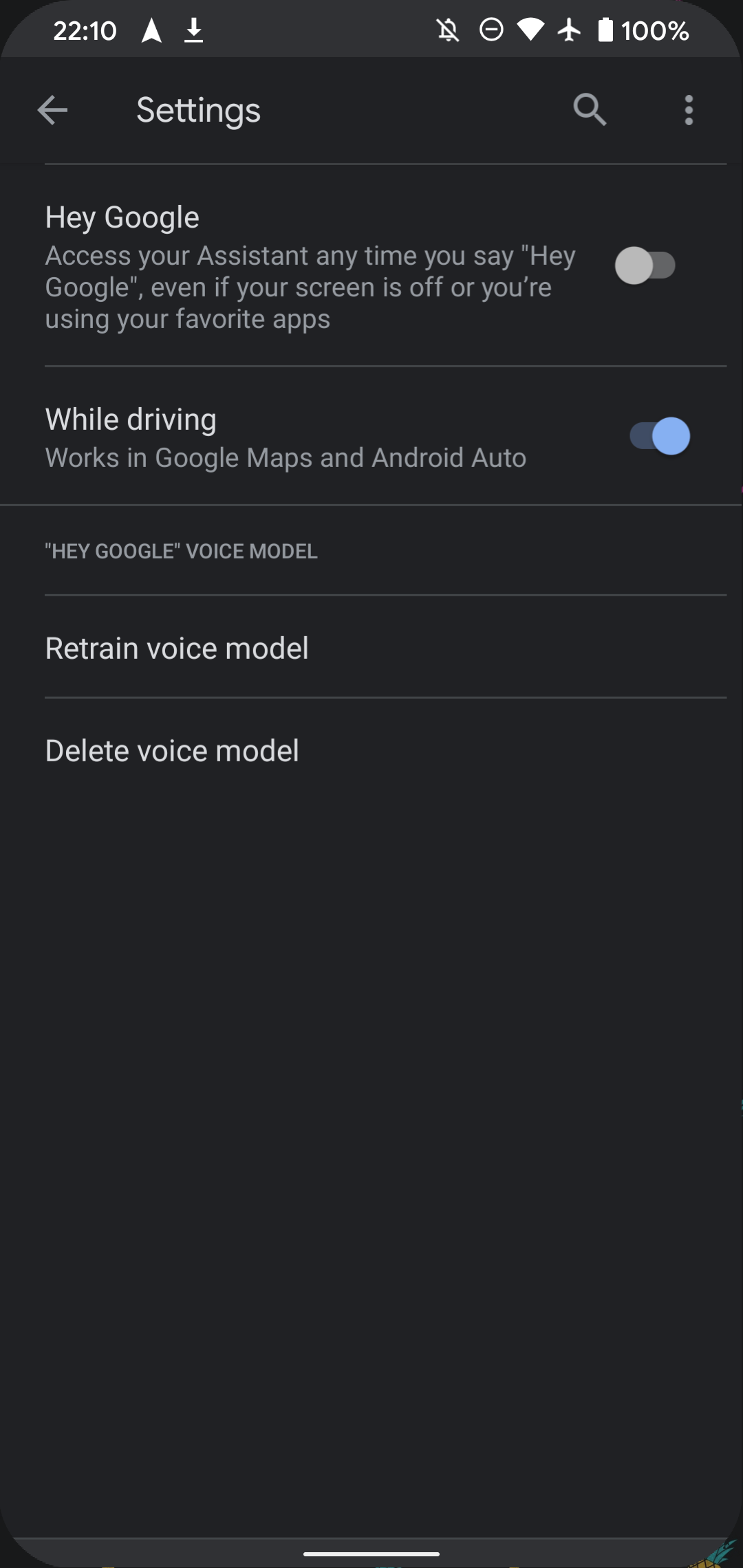This image is a screenshot from a smartphone, displayed in a vertical rectangle with a black background.

At the top in white text, the time is shown as "22:10." To the right of the time, there is an up arrow icon indicating location services are active, followed by a down arrow with a line under it, representing a download symbol. Notifications are turned off, Do Not Disturb mode is enabled, and the device is connected to Wi-Fi. Airplane mode is activated, and the battery level is at 100%.

Directly below this status bar, there is a navigation arrow to go back, a heading labeled "Settings," a search bar, and an options menu represented by three vertically-aligned dots.

The following section features the text "Hey Google: Access your assistant anytime you say 'Hey Google,' even if your screen is off or if you are using your favorite app." This option is toggled off.

Beneath that, it reads "While driving: Works in Google Maps and Android Auto." This option is toggled on. Further below, the text "Hey Google Voice Model" appears, along with options to "Retrain Voice Model" or "Delete Voice Model."

The rest of the screen remains blank, maintaining the black background.